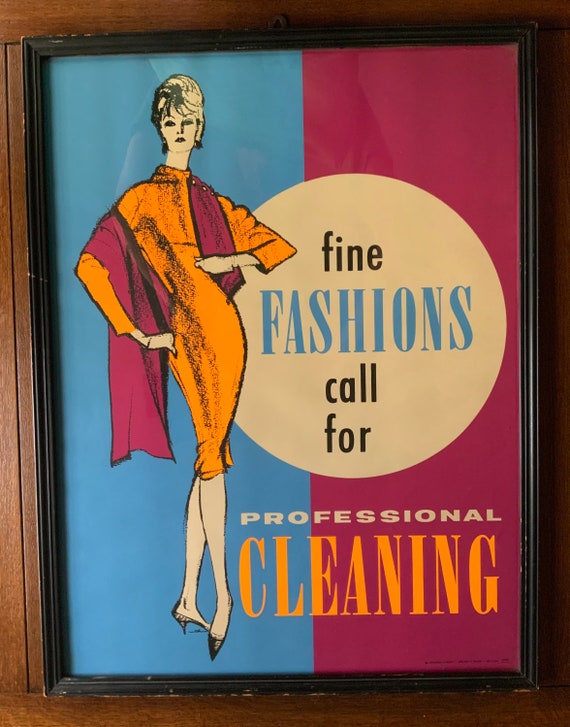This image captures a close-up of a framed vintage advertisement poster for dry cleaning services. The poster is divided vertically into two distinct sections: a robin egg blue left side and a fuchsia right side. Dominating the left side is a detailed vintage illustration of a model, likely from the 1950s, adorned in an orange knee-length long-sleeved dress, paired with a wide magenta shawl that drapes around her neck and extends down to her knees. The model's ensemble is completed with pointy black high heels and a poofy hairdo. In the center of the poster, a large white circle contains the text "Fine Fashions Call 4," emphasizing the retro theme. At the bottom, in bold lettering, the poster proclaims "Professional Cleaning," with the word "Cleaning" highlighted in large yellow letters, matching the color of the woman's dress. The advertisement is encased in an aged, thin black frame, marked by noticeable scratches along the edges, and is mounted on a wooden wall that peeks through slightly behind the frame, adding to the vintage charm of the piece.